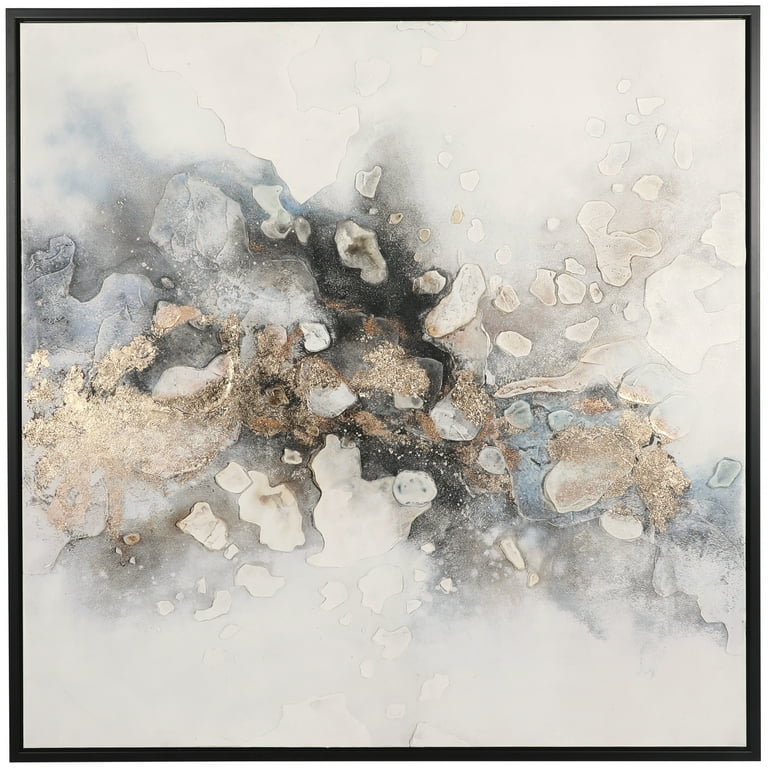The image is an abstract multimedia artwork enclosed in a thin black frame. The centerpiece of the artwork presents a striking, mottled appearance with a mixture of colors including black, gray, gold, light blue, and light beige. This central area has a dynamic, wave-like form, concentrating more gold and black hues in its core, while the outer regions feature lighter shades of blue and gray, ultimately transitioning into a predominantly white haze. Spanning across this scene are delicate, irregular shapes that resemble small crystal rocks or fragments, appearing as though they are cascading or falling gently down the surface. The overall texture is a mix of grainy, sandy patches, distinct from the smoother crystalline forms. The majority of the painting avoids defined brushstrokes, instead exhibiting a natural flow reminiscent of water droplets or smoke, creating an ethereal, soothing atmosphere.